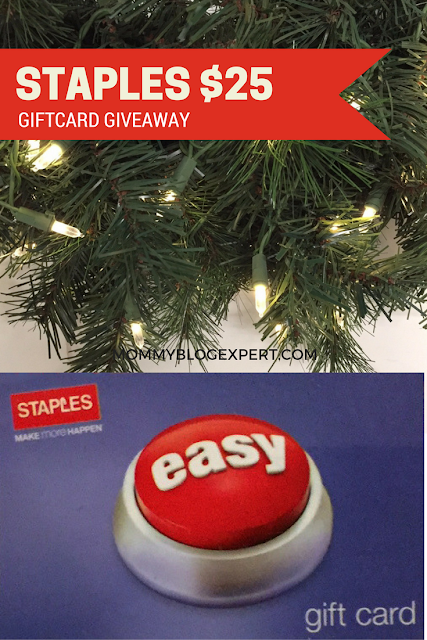This image features a Staples advertisement divided into two distinct sections. 

The top-half prominently displays a close-up of a Christmas tree, intricately adorned with golden lights that twinkle amidst the dense green needles. A vibrant red banner spans across the photograph, boldly proclaiming in white, uppercase letters: "STAPLES $25." Below this, the text "GIFT CARD GIVEAWAY" is also presented in white uppercase letters but in a smaller font. At the very bottom of this section, though slightly challenging to read, the black text "MOMMYBLOGEXPERT.COM" is visible.

The bottom section of the image also advertises Staples, set against a purple background. In the upper-left corner resides the Staples logo—a red rectangle with the word 'Staples' in white. Below the logo, there is a motivational phrase where the first word "MAKE" is clear, the following word is blurry yet appears to be "MORE," and the final word in bold white uppercase letters states "HAPPEN." Dominating this section is a large button colored light gray with a red center. Across the center, in white text, it simply reads "EASY." In the bottom-right corner, the text "GIFT CARD" is displayed.